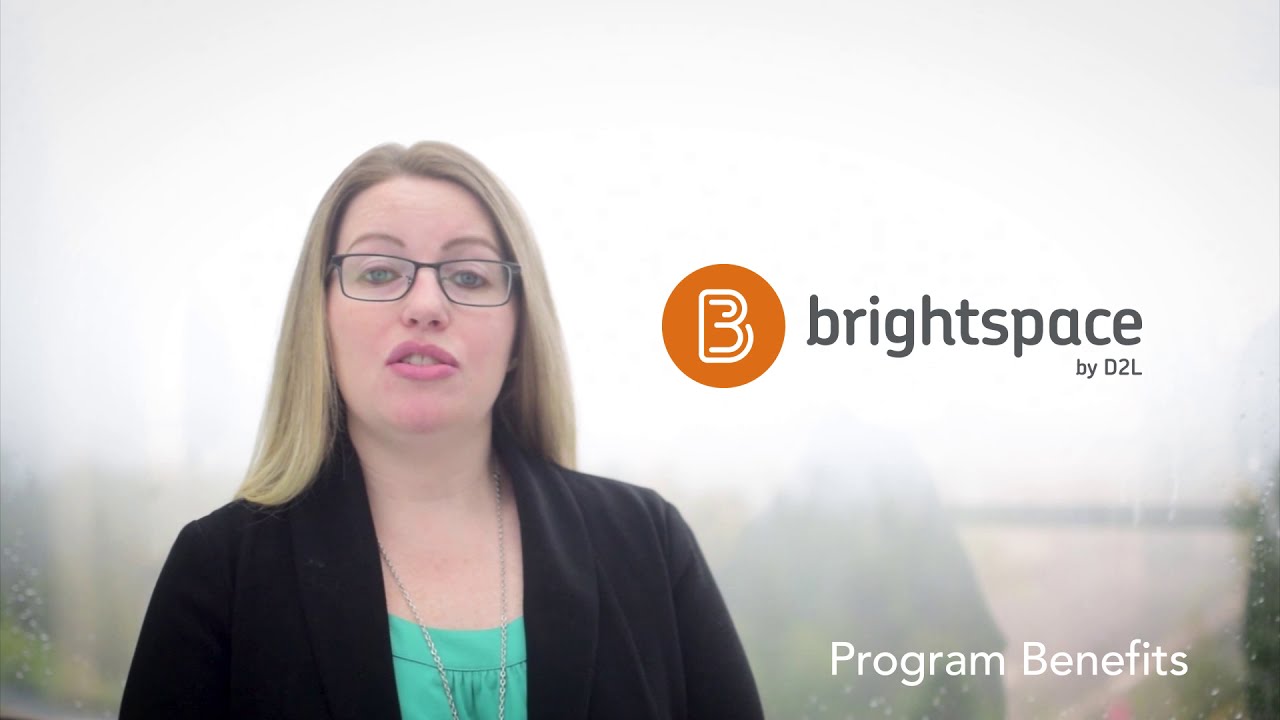The image appears to be a still from a video or possibly a business card, background for a website, or an advertisement. Central to the image on the left-hand side is a Caucasian woman seen from the bust up. She has long blonde hair cascading below her shoulders, with some dark streaks mixed in. She is wearing rectangular, dark-rimmed glasses, her eyebrows raised, and blue eyes, giving the appearance of speaking due to her open mouth revealing her top teeth. She is dressed in a black jacket over a green (or teal) top, accessorized with a long silver necklace.

In the background, which is somewhat faded and appears to show trees, the top part of the image is whited out. On the right side of the image, midway down, there is a prominent orange circle featuring a graphic of a white bee. Adjacent to the circle, the words "Bright Space" are written in black with "By D2L" beneath it. In the lower right corner, written in white, are the words "Program Benefits."